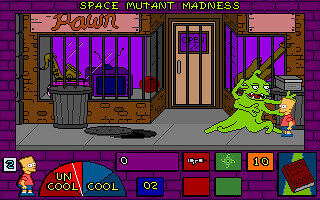This is a detailed screenshot of a video game inspired by The Simpsons, titled "Space Mutant Madness." The setting features a cartoon-like shop in the background with the shop sign prominently displaying "Space Mutant Madness." To the left, there is a trash can on the sidewalk with oil spilled in front of it, barred windows showcasing various items like a TV, a tuba, and a guitar inside a pawn shop. 

On the right side of the image, Bart Simpson stands facing a grotesque green monster. Bart is easily recognizable with his square-shaped head, yellow skin, red t-shirt, blue shorts, and blue shoes. The monster, with green tentacles forming from its body, has four outstretched arms and its mouth slightly open, revealing pointed teeth, as it confronts Bart.

At the bottom of the screenshot, a menu bar is displayed, featuring a "cool" to "uncool" scale and other game stats, including numbers, a book symbol, and what appears to be a needle symbol. To the right, more buttons or menu options can be seen, emphasizing various game functionalities.